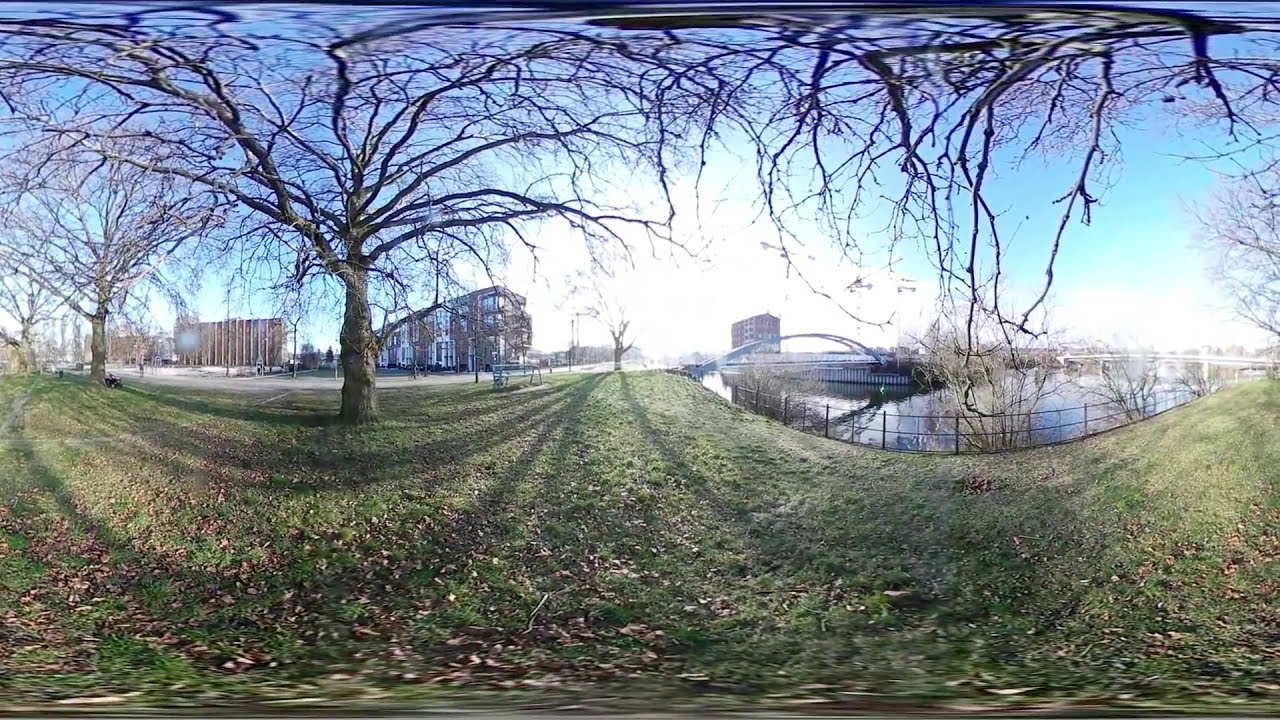This image is a wide panoramic, fish-eye view of a long park adjacent to a body of water, featuring distinct urban and natural elements. The curved perspective reveals a grassy area speckled with multicolored green grass and scattered brown leaves, indicating a change in seasons. This green expanse curves downward and upward across the frame, leading to a large body of water on the right, framed by a railing. Multiple arched bridges span the water, their structures reflected in the calm surface below.

On the left side, towering trees with bare, expansive branches dominate the scene, their presence casting intricate shadows despite the absence of leaves. In the distance, similar leafless trees contribute to the park's late-autumn or early-winter atmosphere. Beyond the tree line, a cluster of multi-story brick buildings stands, characterized by numerous windows that suggest residential or institutional use, potentially apartment complexes or schools.

The sky above is a mix of clear blue and patches of cloud, illuminated by bright sunlight that creates vivid contrasts and occasionally washes out finer details. The overall setting exudes a serene, daylight atmosphere, capturing the tranquil yet dynamic essence of the urban park and its surrounding environment.